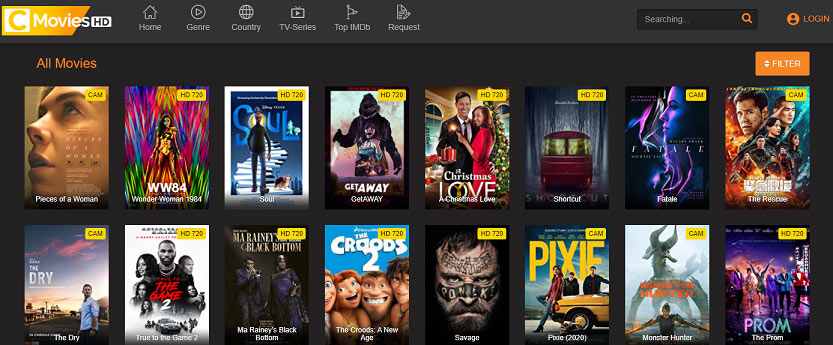The image showcases a web page designed for movie purchases with a structured and organized layout. The background is a dark gray, providing a sleek contrast to the elements on the screen. At the top, a menu bar, also in dark gray, spans the width of the page. On the far left, there's a logo displaying the letter 'C' followed by the text "Movies HD."

The menu bar features several options, each accompanied by an icon above the text: 
- "Home" 
- "Genre" 
- "Country" 
- "TV Series" 
- "Top IMDB" 
- "Request"

On the right side of the menu bar, there is a search bar labeled "Searching" with an orange magnifying glass icon inside it. Further to the extreme right is an orange "Login" button.

Below the menu bar, there is a table titled "Top Movies," highlighted in orange. This table is segmented into rows showcasing multiple movie thumbnails. The top right corner of the table features a filter option with an orange button labeled "Filter." The table displays two rows of movie thumbnails, with eight movies per row. Some of the visible titles include "A Christmas Love" and "Shortcut," while the others are unclear or unreadable.